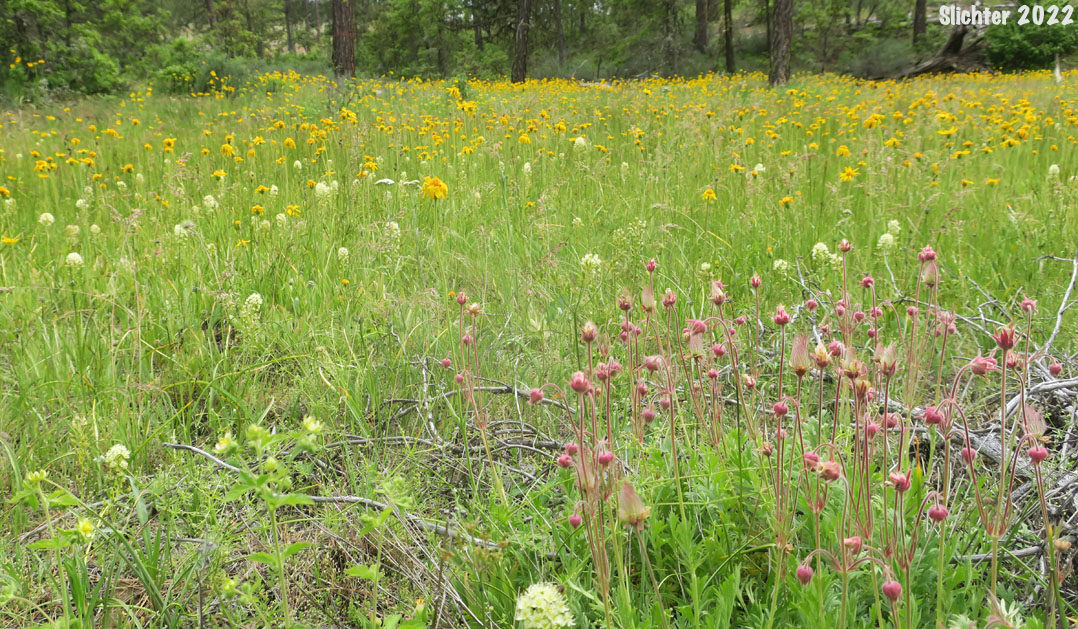This image captures a lush, open field abundant with a diverse array of wildflowers on a semi-sunny day. The foreground is adorned with tall wildflowers, some reaching past hip height. The field is a vibrant tapestry of colors dominated by green hues, ranging from dark to light shades. Yellow flowers are scattered generously throughout, while pink long-stem buds and white flowers are also visible, adding to the rich diversity of the flora. Small grayish-tan twigs are interspersed among the grass. The field stretches into the distance where it meets a denser collection of trees and vegetation, creating a verdant boundary. In the upper right corner, there is a watermark that reads "Fletcher, S-L-I-C-H-T-E-R, 2022," subtly marking the photograph. This daytime capture beautifully highlights the natural beauty and varied colors of this wildflower-dotted field.